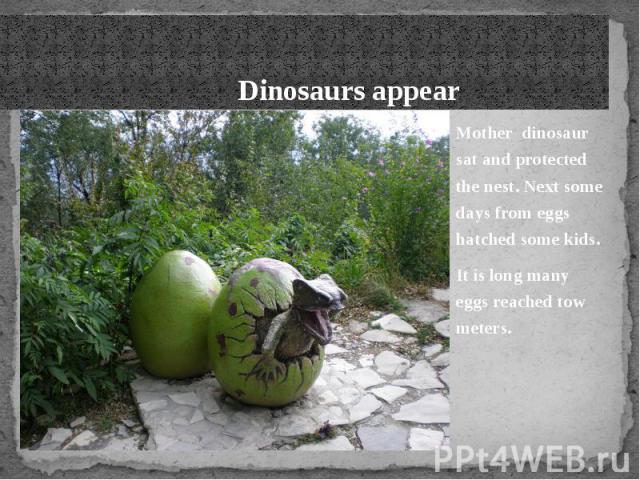This image appears to be part of an educational PowerPoint presentation, possibly a digital slide meant to discuss dinosaur reproduction. Encased in a stone-like border with a dark gray, textured top bar, the slide's overall design suggests a prehistoric theme. At the top right, text reads: "Dinosaurs appear," followed by a brief narrative describing a mother dinosaur protecting her nest and eventually, baby dinosaurs hatching from the eggs.

Dominating the left side of the slide is a detailed image situated on a rough, stone pathway. Two large, green dinosaur eggs rest on the uneven path; one egg is cracked open, revealing an emerging miniature dinosaur with its paw gripping the shell and its mouth open, as if roaring. Behind these eggs, lush greenery including bushes, trees, and some flowers adds depth to the scene.

Further to the right side, additional text supplements the narrative: "Mother dinosaur sat and protected the nest. Next, some days from the eggs hatched some kids. It is long, many eggs reached to meters." At the bottom right corner, a watermark displays the URL "ppt4web.ru," indicating the source. The overall color palette includes varying shades of gray, white, black, and green, enhancing the prehistoric and natural atmosphere of the presentation.